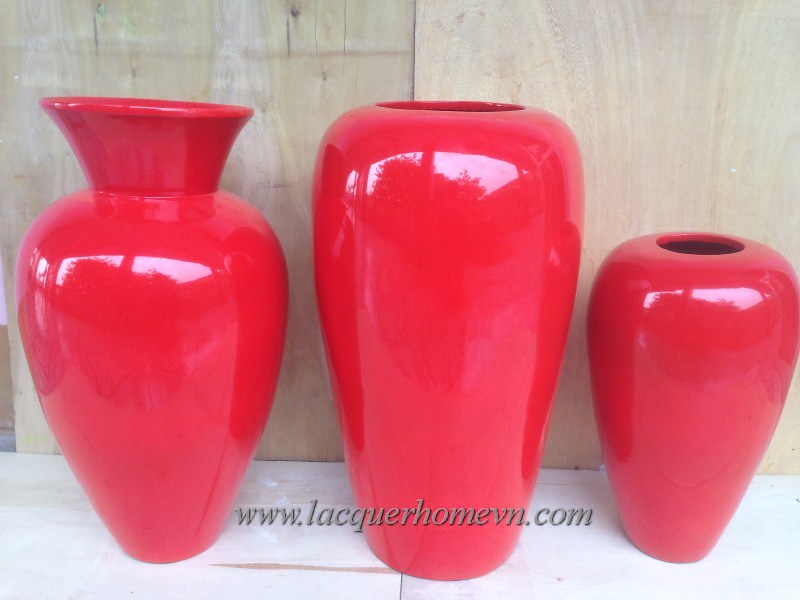In this image, we see three bright red flower pots of varying shapes and sizes arranged on a white tile floor. The background features a light brown wooden cupboard, creating a cozy, homey atmosphere. On the left is a uniquely heart-shaped flower pot with a narrow base that widens dramatically towards the top, ending with a cone-like opening. The center pot is the largest, presenting an oblong, cylindrical shape with a notable taper towards the bottom and a distinctive cut-out in the middle. To the right is the smallest pot, which is thin at the bottom and wider at the top, creating a rounded, compact appearance. The surfaces of the pots are reflective, adding to their vibrant and eye-catching appeal. A watermark, "www.lacourhomevn.com," suggests that the image is likely from a home decorating website, possibly used for advertisement purposes.